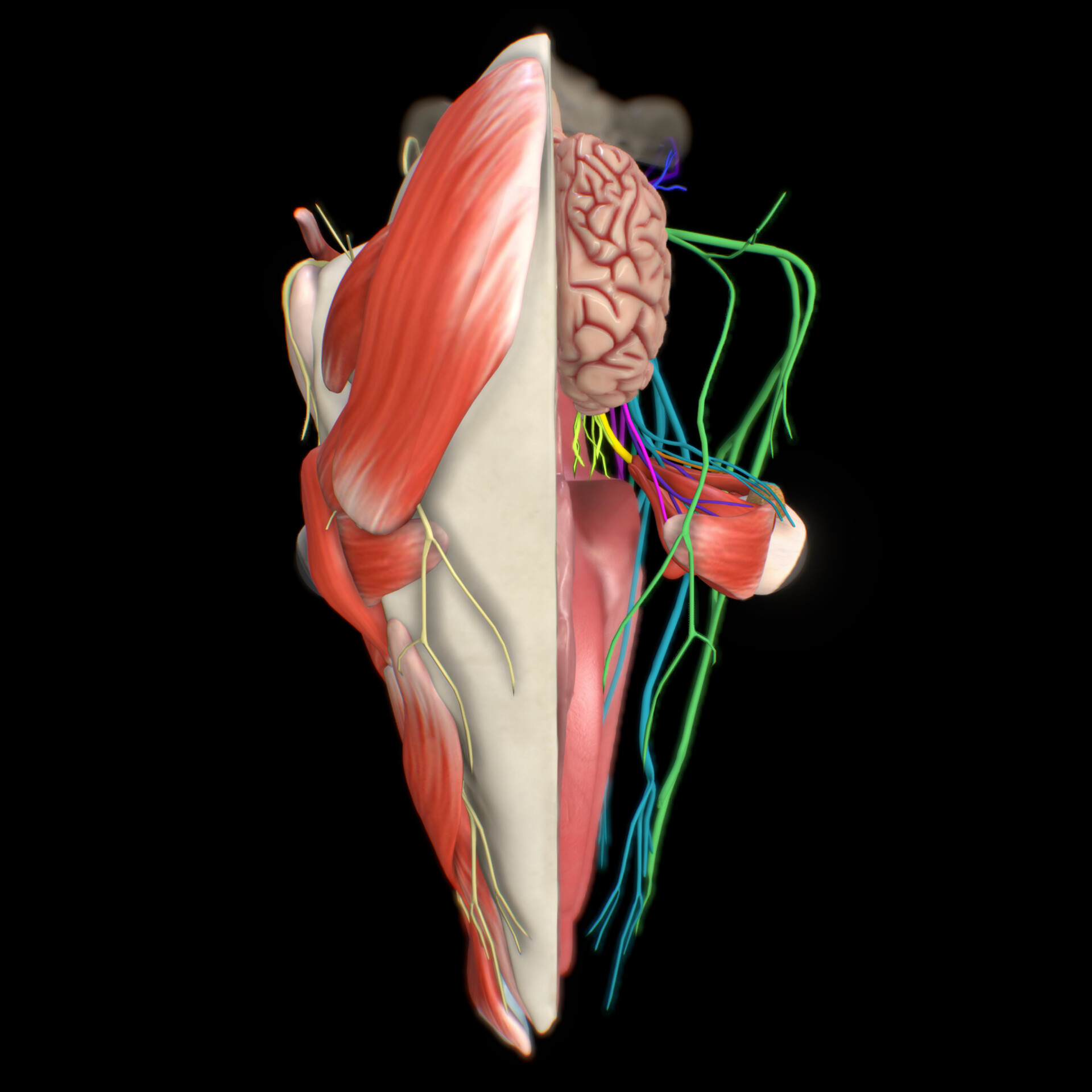The image appears to be a detailed dissection of an animal, possibly a mouse, likely framed for a medical textbook. At the top, a mouse's head is identifiable with its ears protruding. The dissection splits vertically down the middle, revealing distinct anatomical structures on either side. 

On the right side, a rounded object, likely a brain, is visible. Several prominently colored veins or nerve-like structures extend from the brain: green, magenta, yellow, and aqua. Below the brain, a reddish shape with a rounded white piece, possibly connective tissue, appears to be an anchor point for some of these veins. 

The left-hand side depicts muscles and tendons in a spectrum of red, pink, and white hues. These structures interconnect intricately and are attached to what might be a piece of bone. Light green vein-like structures emanate from the muscles, potentially indicating tendons. The entire composition is set against a stark black background, enhancing the visibility of the anatomical details in the image.